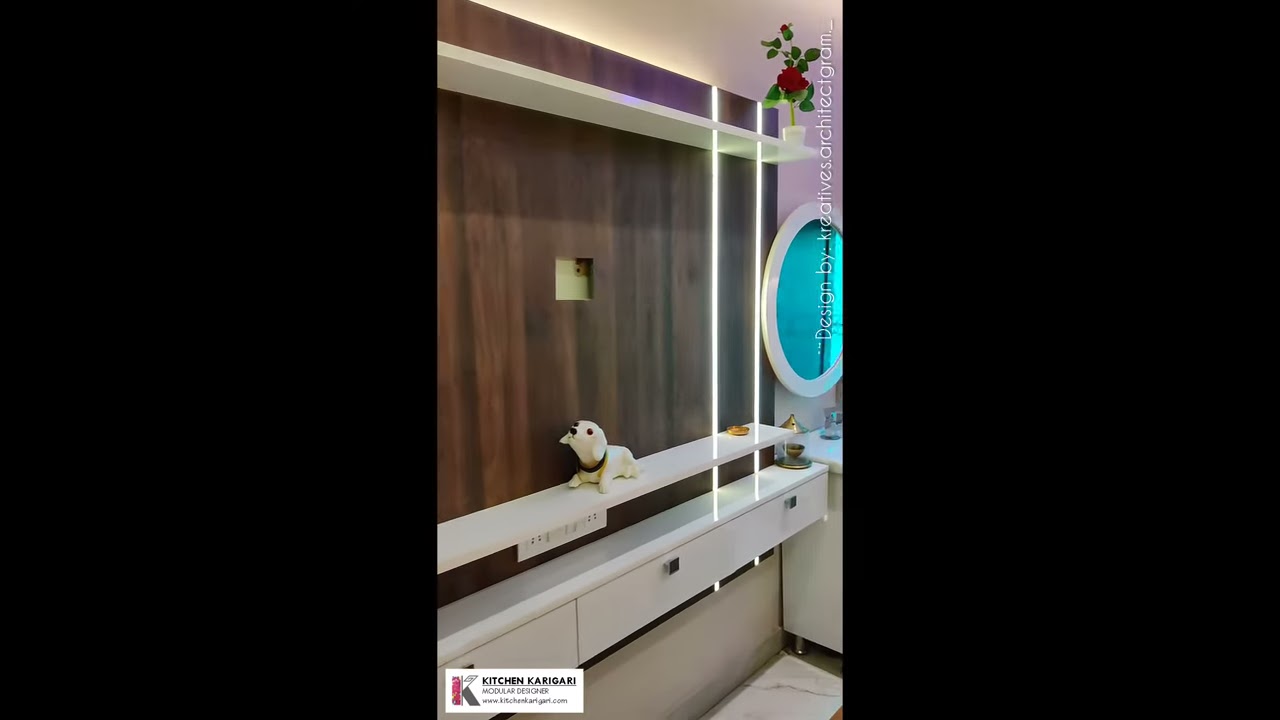The image appears to be a digital snapshot from a phone, featuring a small room with modernist design elements. Central to the photograph is a wall of dark wood or vinyl paneling, with contrasting white shelves. The topmost shelf spans the length of the wall and supports a blooming plant with vibrant red flowers in a small white pot. Below this, a second shelf holds a stuffed white dog toy, positioned prominently in the center. Directly beneath this, a third shelf supports a set of white drawers with black handles. An oval mirror with a white frame, which might be turquoise or reflective, is affixed to the wall on the left, adding depth to the setup. To the right of these shelves are two vertical, cylindrical white lights that brighten the scene. A small, barely legible white sign located in the lower right corner hints at branding, featuring the partial text "Designed by K dot Architect Graham underscore." The meticulous arrangement and sleek design suggest a room that could be part of a bathroom or a display area, bathed in a clean, minimalist aesthetic.